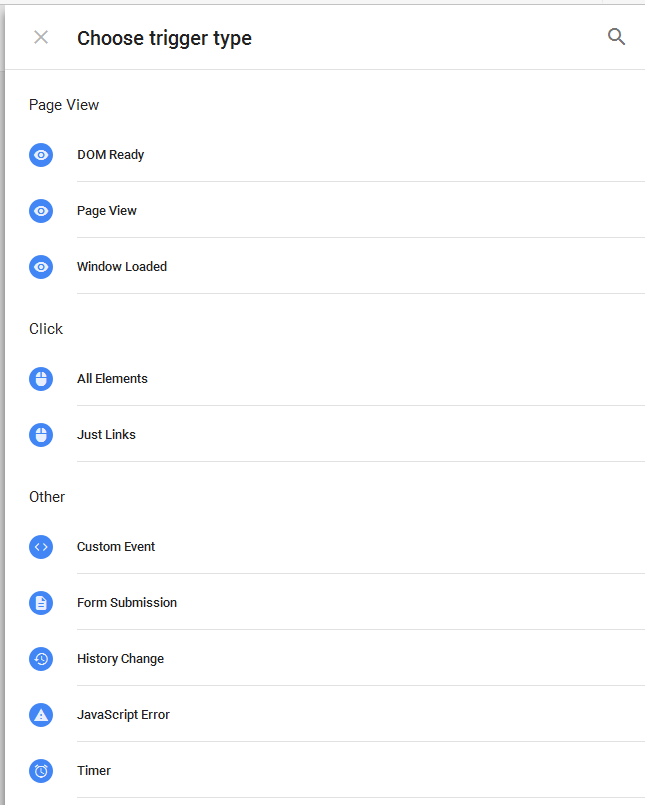This is a detailed screenshot of a settings window within an application, showcasing a layout and various options available to the user. The window has a clean white background with a faint light gray shadow along the left and top edges, adding subtle depth to the interface.

At the top, the header features a muted light gray 'X' icon on the left side, followed by a bolded black text that reads "Choose Trigger Type." To the far right of the header, there's a medium gray magnifying glass icon. The header is distinctly separated from the main body by a thin light gray line.

The body of the window is organized into several sections with their own titles and icons. At the top left, in medium gray text, it says "Page View." Underneath this title, there are three blue circular icons, each with a white eye symbol inside. Accompanying these icons to the right, concise yet informative labels are present in small-sized, bolded black text: "DOM Ready," "Page View," and "Window Loaded." Each of these items is divided by thin light gray lines, maintaining clear visual separation.

Moving further down, the next section is titled "Click," also in medium gray text. Below this title, there are two blue circular icons, this time with white mouse symbols. These are labeled, respectively, as "All Elements" and "Just Links," again separated by thin light gray lines.

At the bottom left, another section title, "Other," is displayed in medium gray text. Beneath this heading, five blue circular icons are presented, each showcasing different white icons and labeled accordingly from top to bottom: "Custom Event," "Form Submission," "History Change," "JavaScript Error," and "Timer." The consistent use of thin light gray lines continues to ensure clarity and separation between each of the labeled options.

Overall, the interface is neatly organized, visually calming with a consistent use of colors and icons, facilitating easy navigation and understanding of the various settings available within the application.